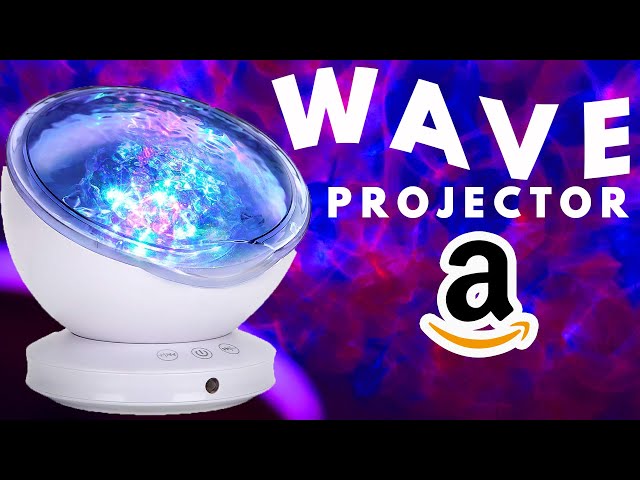The image showcases a white wave projector prominently placed against a dynamic red and blue background with a marble-like pattern. The wave projector, resembling a white spherical bowl atop a round platform with three buttons, is depicted on the left side of the image. It features a plastic lid that appears to be projecting light, creating the colorful wave effect in the background. The advertisement includes bold white text, with 'WAVE' in large capital letters that follow a wave pattern and 'projector' written beneath it in smaller text. The black and yellow Amazon logo is located below the text, indicating that the product can be purchased from Amazon. The photo is horizontally oriented, framed by black stripes along the top and bottom edges.